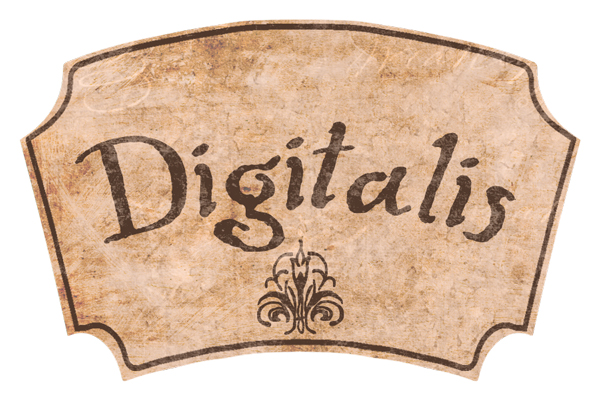The image features a single, irregularly shaped sign with an arched top and inwardly curved corners, resembling a rectangle with rounded cut-off edges that bends slightly downward. The background of the sign is a washed brown and white color, with darker brown edges that give it a rustic, textured appearance akin to aged newspaper print. Dominating the center of the image is the word "Digitalis" written in a dark brown, almost handwritten cursive font. Beneath the text is a matching fleur-de-lis symbol, also in dark brown, which complements the overall design. The entire sign is outlined in a dark brown marker-like border, adding to its vintage and handcrafted feel. There are no additional elements or details to indicate the context, such as whether it is an advertisement, a web page, or a flyer.